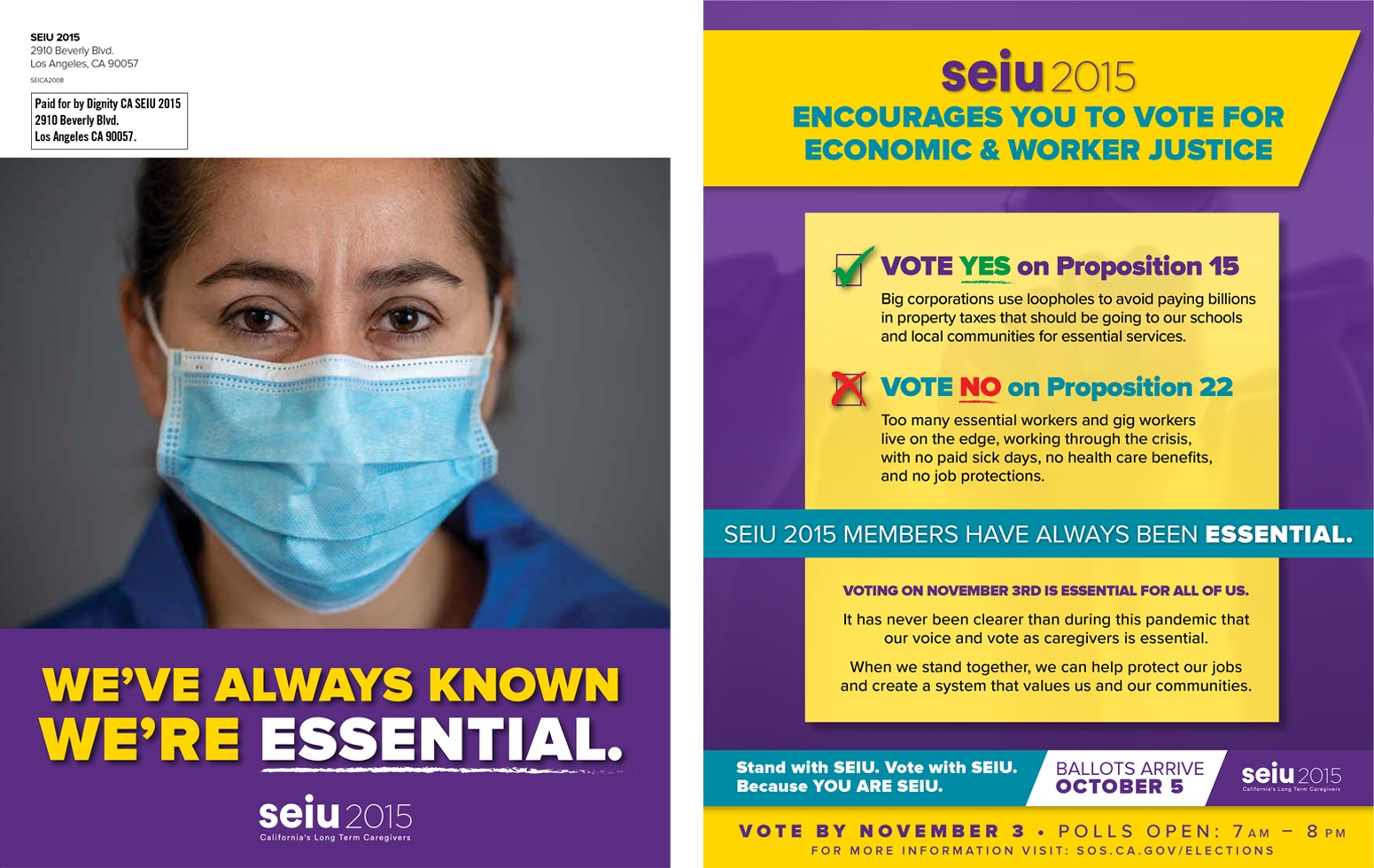The promotional flyer from SEIU, 2015, is aimed at California's long-term caregivers, urging them to vote for economic and worker justice. The content heavily focuses on endorsing a "Yes" vote for Proposition 15, which targets closing corporate loopholes and ensuring billions in property taxes support schools and essential local community services. It also promotes a "No" vote on Proposition 22 to protect worker rights.

The flyer is visually striking with a dominant color palette of purple and yellow. The left side of the flyer features an image of a Hispanic woman wearing a blue surgical mask, directly engaging the viewer with her gaze. The text emphasizes the urgency of voting, noting key dates for receiving and submitting ballots, and provides resources for more information, such as the link to the California Secretary of State's elections website (sos.ca.gov/elections). 

Overall, the flyer is a call to action for caregivers, encouraging them to exercise their voting rights to promote justice and fairness in their industry and beyond.